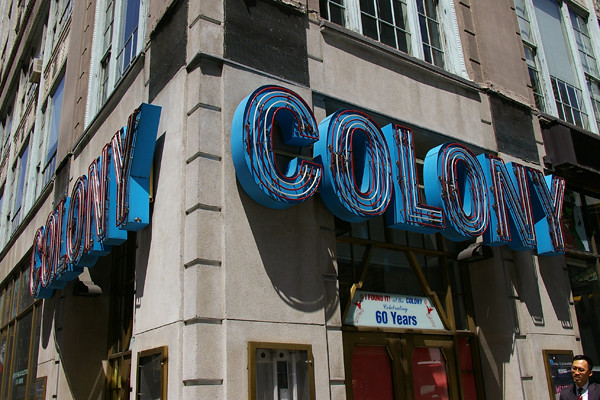The image depicts a close-up view of a large, multileveled, stone gray building on a street corner, exuding an urban city vibe. The building's façade is adorned with white-framed windows, scattered evenly up its sides. Prominently, a blue neon sign bearing the word "Colony" is affixed to both sides at the base of the corner. The neon tubing adorning the large, block letters is styled in red and white, although the lights appear dormant in the daylight. Directly below each "Colony" sign, a smaller white sign proudly announces "Celebrating 60 Years." Additionally, red doors can be seen below the signs, suggesting an entrance.

On the sidewalk beside the building, an Asian man is walking, captured in the lower right-hand corner of the image, with only his head and shoulders visible. Near the doors and along the walls of the corner, built-in cases for posters are found, with one case behind the man displaying a poster while the others remain empty. The overall setting hints at a common urban city scene, potentially indicating the establishment as a movie theater or similar venue.